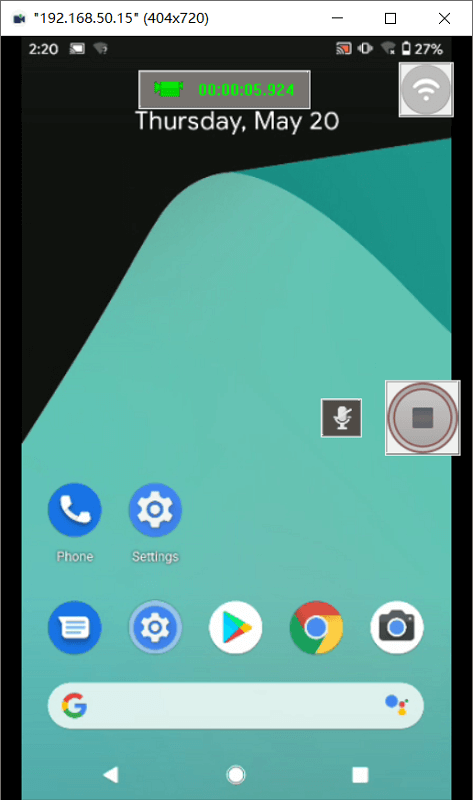This image is a detailed screenshot of a smartphone’s screen. At the top-left corner, the time is displayed as 2:20 PM. The top-right corner shows the battery level at 27% and includes an icon indicating the network connection strength. Prominently in the top-middle, green text signifies an ongoing recording, displaying a timer that reads 00:05.924 with a small green camera icon adjacent to it. The date, Thursday, May 20th, is clearly visible just below this section. To the right of the date, a microphone icon is shown crossed out, indicating that the microphone is muted during the recording. Adjacent to this is a stop button, ready to halt the recording when pressed. Toward the bottom of the screen, several app icons are visible, including Phone, Settings, and Text Messaging, along with a Google search bar at the very bottom.